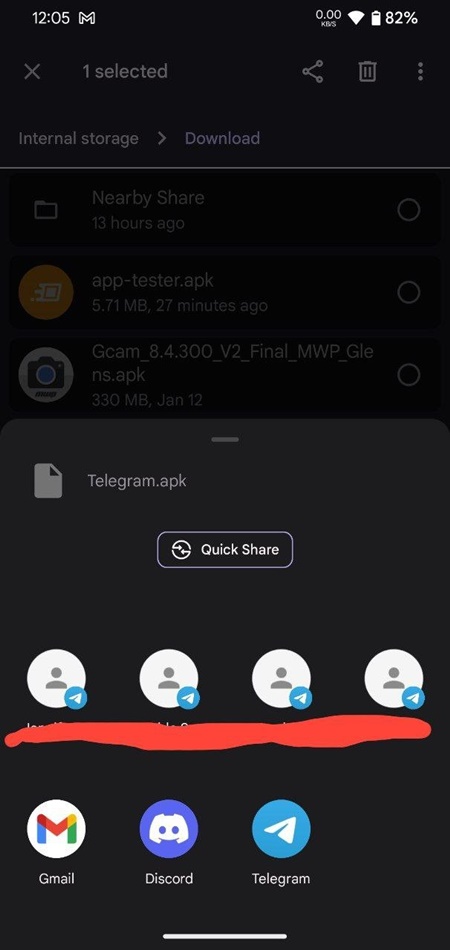The image is set against a black background and appears to be a screenshot from a cell phone. In the upper left corner, the time is displayed as "12:05" in white text. The "M" icon from Gmail is visible near the top. On the upper right corner, both the Wi-Fi icon and the battery icon are displayed, with the battery level showing 82%. 

Below, a dimly lit search bar contains the text "one selected". Underneath, it reads "Internal storage" with a right arrow indication. Beneath this, there is an option labeled "Nearby Share" accompanied by a file icon on the left and a timestamp of "13 hours ago" below it. There is an orange circle icon, and to its right, the text "AppTester.apk" with a file size of "5.71 MB" is indicated, along with a timestamp of "27 minutes ago". At the very bottom of the screen, there is a white-outlined action button labeled "Quick Share".